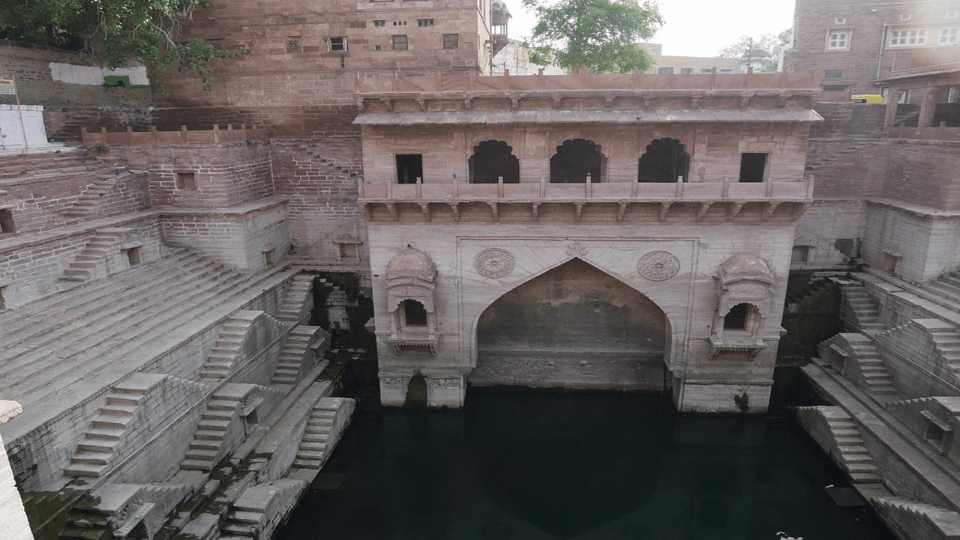The photograph captures an ancient, grand building made of worn brick and stone, showcasing a timeworn aesthetic with classical architectural details. The central structure, prominently featuring a domed area, is flanked by staircases that ascend from both the left and right sides to various flat levels. The building's façade includes windows that protrude outward and several smaller windows near the top. 

Taken outdoors in natural daylight, the image reveals a tree and sky in the background, suggesting the setting is under an open sky. There's also a dark green body of water, possibly filled with algae, at the base of the building. The overall scene has an old-world, almost Roman or gladiatorial atmosphere, imbued with lively details that suggest a bustling area. The photograph, full of vibrant and lively elements, captures not only the ancient architectural beauty but also a sense of historical significance and communal life in the background.